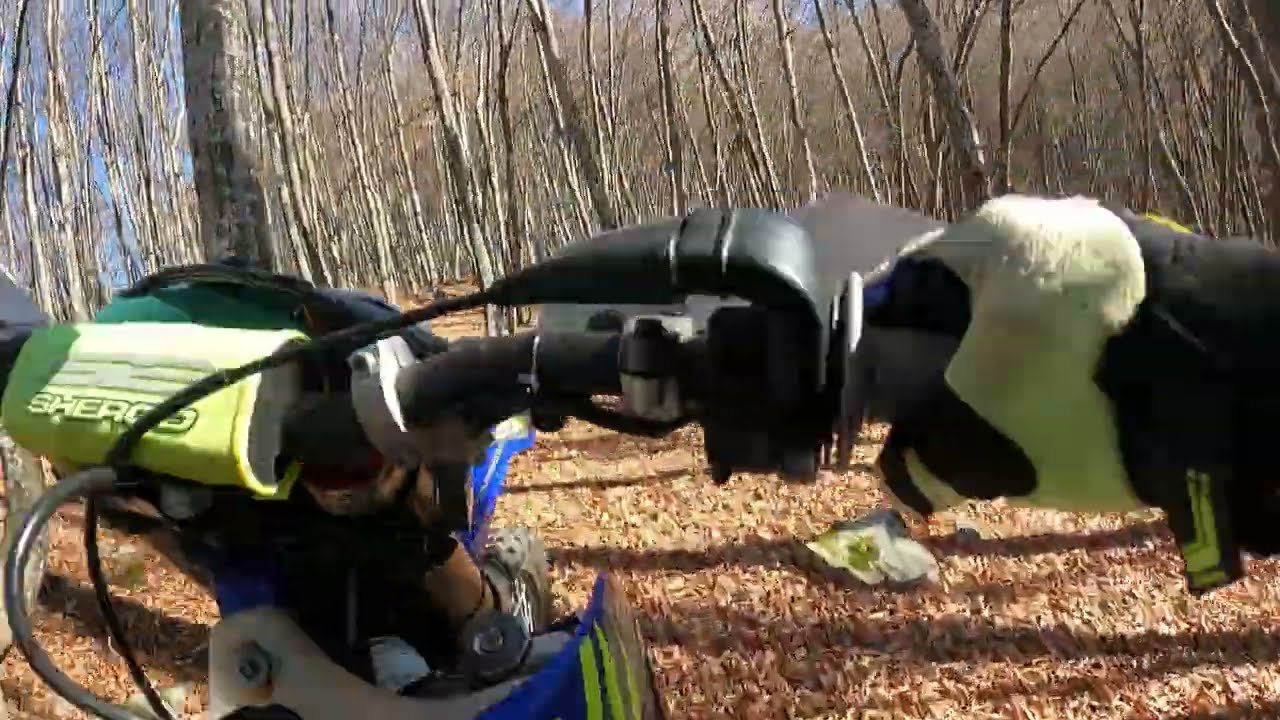The image depicts a person operating a dirt bike in an autumnal or winter woodland setting. The shot, possibly taken from a GoPro, is slightly pixelated and closely focuses on the right handlebar, gripped by a black and yellow-gloved hand. The motorcycle features a mix of black, yellow, blue, and a hint of green. Surrounding the bike, a forest of thin, leafless trees dominates the background, with fallen leaves, dirt, and scattered branches covering the ground. The upper portion of the image provides a glimpse of the sky through the bare trees, suggesting a late-fall or early-winter timeframe.